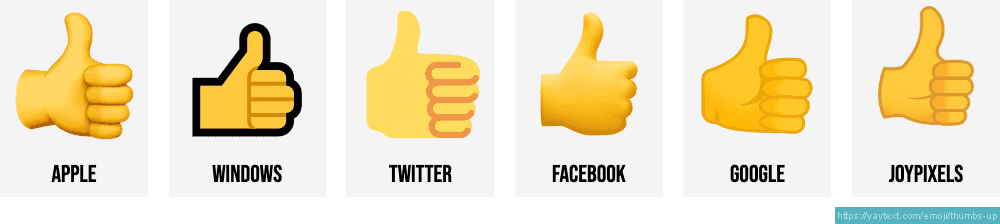This image illustrates the variations of the thumbs-up emoji used by six different social media platforms: Apple, Windows, Twitter, Facebook, Google, and JoyPixels. Each emoji is positioned above its respective platform's name, written in black lettering. All the thumbs-up emojis are a shade of orangish-yellow or goldish-yellow, with slight differences in design. The Windows emoji is distinctively outlined in black. Most of the emojis depict the fingers beside the thumb, and one shows the opposite side of the hand. The background of the image is white, with each emoji set within light lilac-colored rectangles. A small website address, yatext.com/emoji-thumbs-up, appears at the bottom of the image, indicating its source.